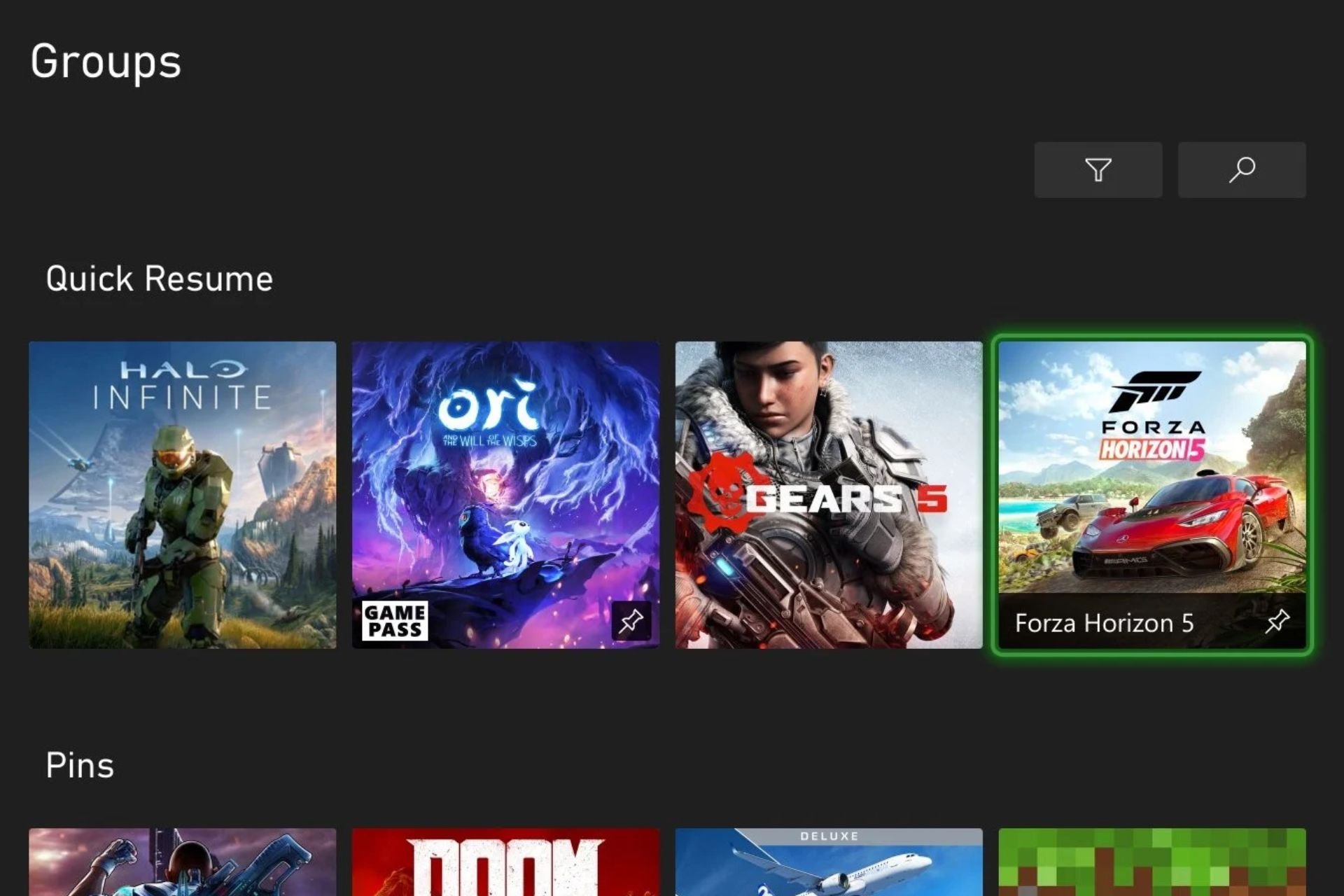This image captures a detailed screenshot, likely from a desktop interface, displaying a curated list of games. At the top of the interface, the heading "Groups" is prominently visible, indicating the organization of the games into various categories. 

Beneath this heading, the games are neatly arranged into groups, with the first group featuring tile icons for four different games:
1. **Halo Infinite:** The icon showcases the game’s distinctive cover art.
2. **Ori:** Accompanied by a "GASP Game Pass" stamp and a pin icon, signaling its availability on Game Pass and its pinned status.
3. **Gears 5:** Displayed with its recognizable game art.
4. **Forza Horizon 5:** Similarly marked with a pin icon next to its tile.

Directly below this set, the word "PINS" appears, indicating a section reserved for pinned games. In this section, there are four additional game tiles partially visible, each about 25% revealed, making some titles difficult to discern:
1. **Minecraft:** Clearly identifiable by its iconic blocky aesthetic.
2. **A game with 'Deluxe' in its title and an image of a plane.**
3. **DOOM:** Easily recognized from the bold typography of its title.
4. **An unidentifiable game, displaying only a character with their back turned, lacking sufficient detail to determine its identity.**

The visual composition and detailing of the interface strongly suggest it is optimized for desktop viewing, providing a structured and categorized presentation of the listed games.